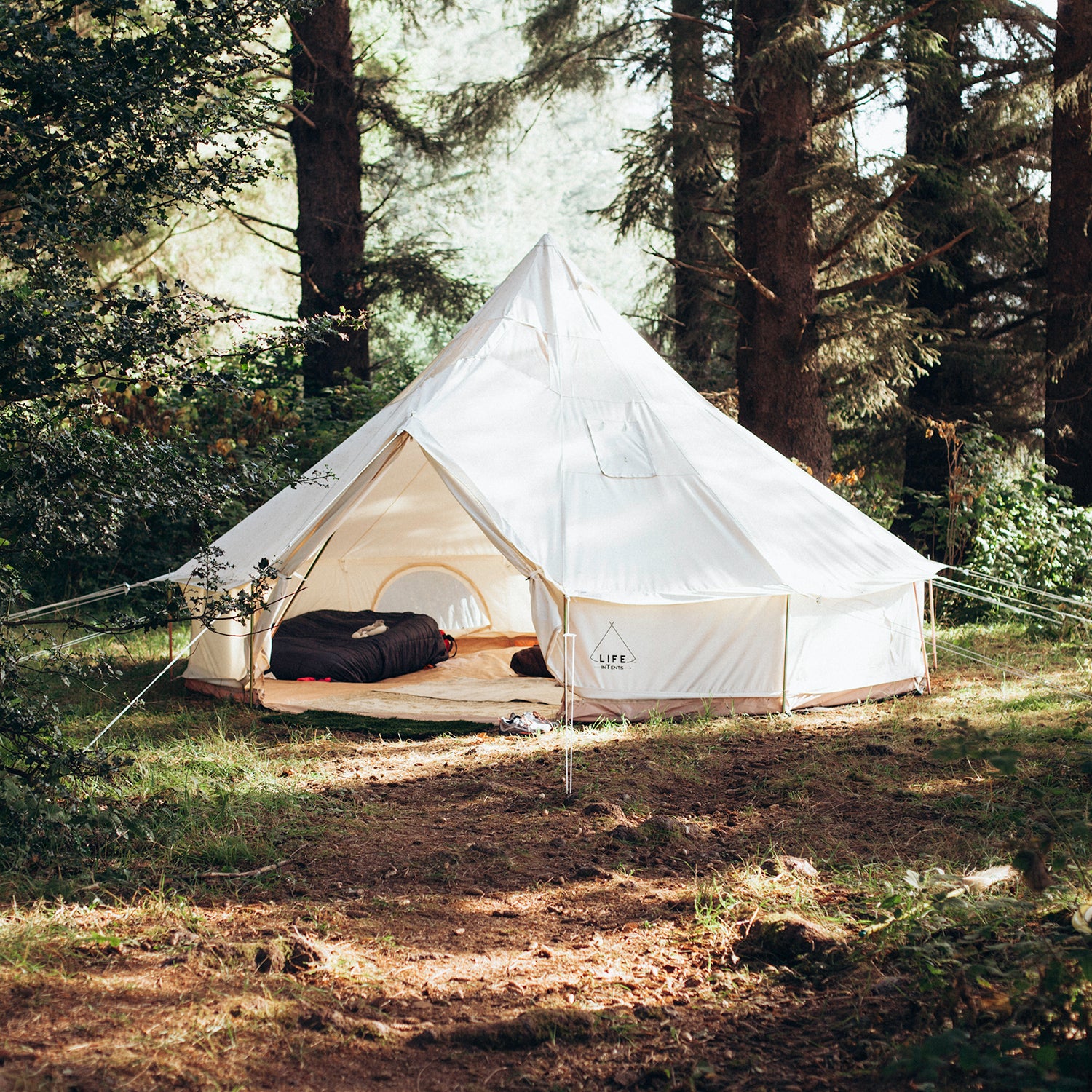This image depicts a sunny outdoor scene in a forested area with tall pine trees. At the center is a large, round, white teepee-style tent anchored firmly to the ground with several support ropes. The tent is situated on a clearing featuring brown dirt and patches of grass. The tent, which has an open door revealing a glimpse of a black object and an air mattress inside, looks spacious enough to sleep four to six people comfortably. Additionally, there are small, zippered windows on the tent and some unreadable small letters printed on it. The shadows cast by the trees and tent contribute to the overall tranquil and inviting atmosphere of the campsite.